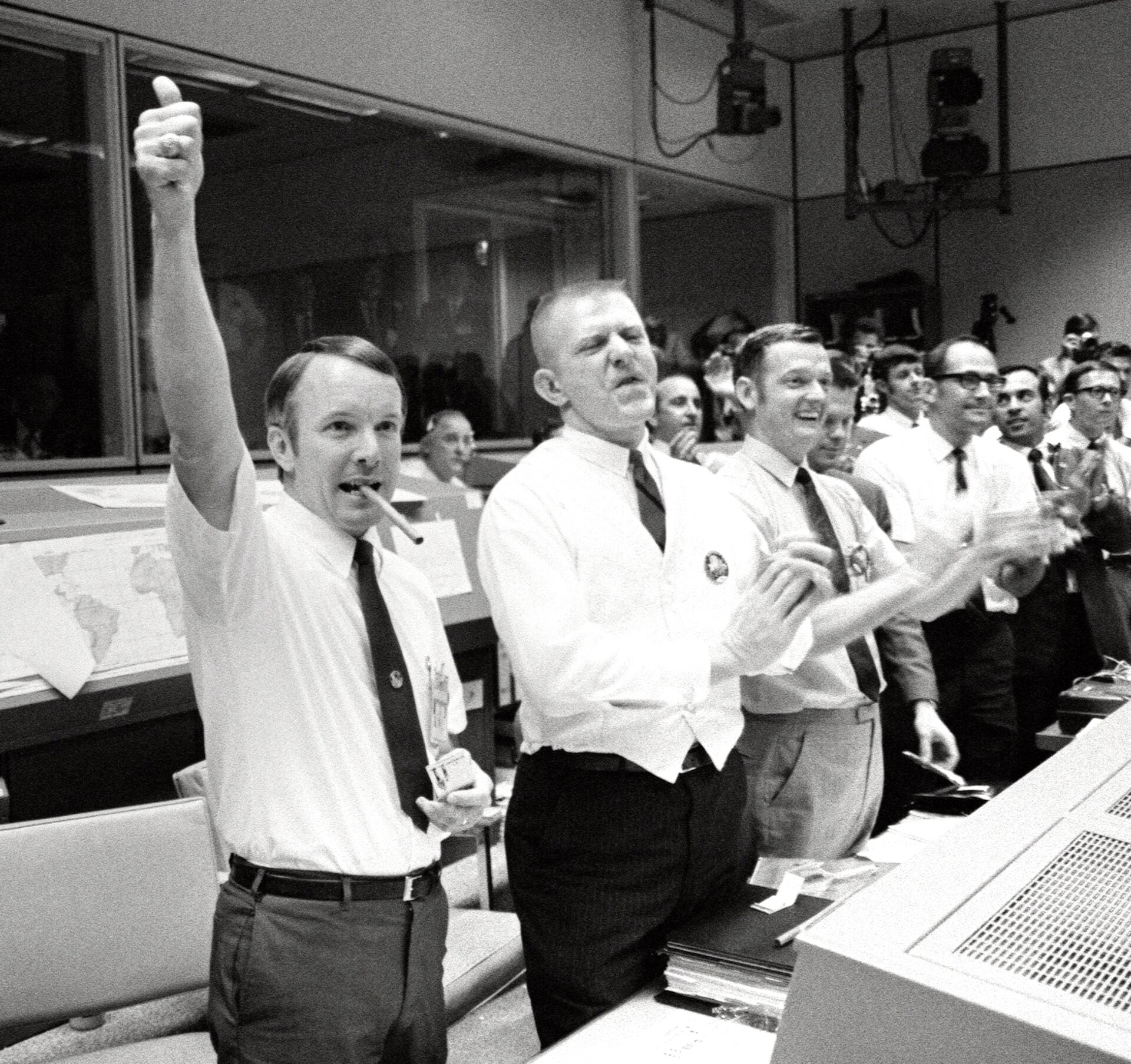This black-and-white photograph captures an energetic moment in the NASA control room, likely from a successful space mission in the late 1960s to early 1970s. The foreground features a row of predominantly white men dressed in white shirts, black ties, and various shades of slacks. The man closest to the camera on the left stands out with his gray slacks, white tucked-in shirt, and thumbs-up gesture, a long cigar poised in his mouth. To his right, another man, with a crew cut and wearing black slacks, claps his hands halfway between a scowl and a smile. Further right, another man with light slacks is enthusiastically clapping, his hands blurred from the motion. All the men are clearly celebrating, looking towards something behind and to the right of the camera. Their joyous expressions and applause suggest a momentous achievement. The background reveals large, dark windows set into a light gray wall, with what seems to be a world map partially visible behind the leftmost man. There is also camera gear hanging from the ceiling in the top right of the frame, adding to the room’s technical atmosphere.